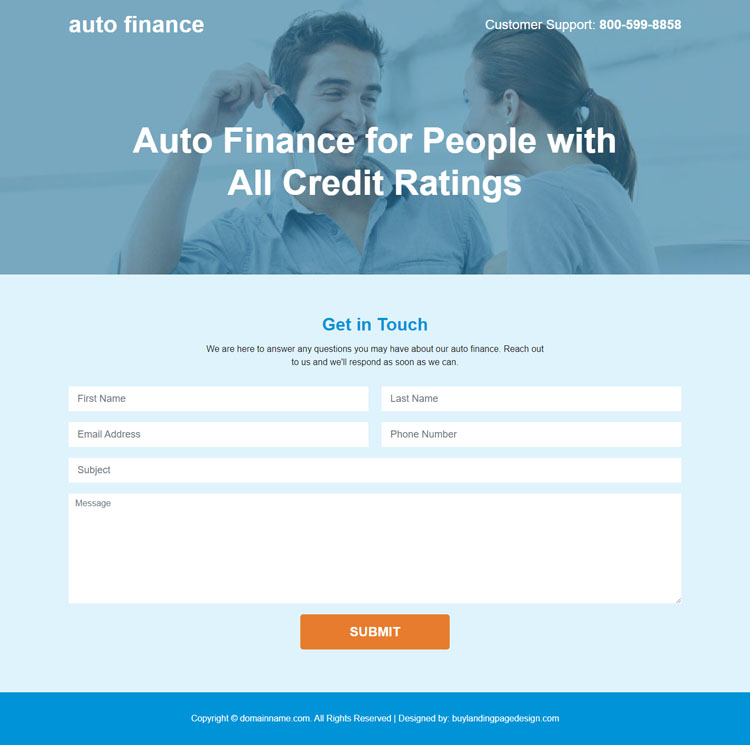This is a detailed descriptive caption for the provided image:

---

The screenshot has a squarish shape and is divided into three sections. The bottom-most section features a very light blue stripe with a copyright notice that reads "© domainname.com." Above this, the middle section displays a large form against a light blue background, though much of the space is unused and dominated by tiny fonts. At the top center of this middle section, there's a heading in blue text that reads "Get in touch." Below it, the form contains fields for first name, last name, email address, phone number, subject, and message. It also includes an orange "Submit" button, which is disproportionately large compared to its small-font text. The form section additionally carries a message in tiny font: "We are here to answer any questions you may have about our auto finance. Reach out to us and we'll respond as soon as we can."

The top section features a background photograph depicting a light-skinned man and woman, both with brown hair and dressed in light blue summer shirts. The man, standing on the left, holds an indiscernible object in his right hand while they both smile at each other. Text overlays the image, with "Auto Finance" in the upper left corner and "Customer Support" along with a phone number in the upper right corner. Prominently displayed across the top section are the words "Auto Finance for people with all credit ratings," indicating inclusivity in their credit offerings.

---